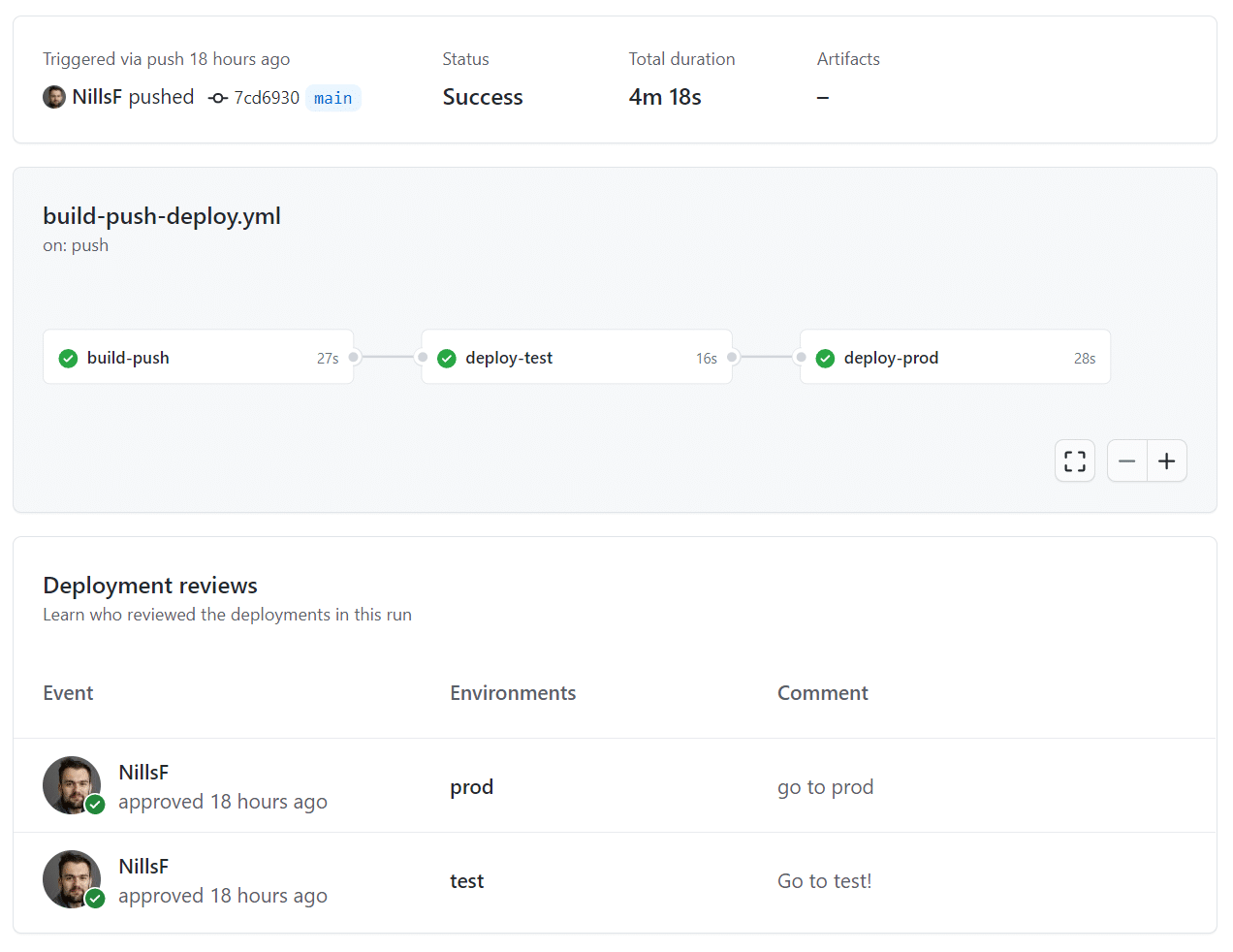Screenshot of a computer screen displaying a build and deployment pipeline interface. At the top of the screen, a status message states, "Triggered via push 18 hours ago." Adjacent to this message, a small icon of a man is visible along with the text "NILS F pushed." The status is marked as "success" with a total duration of 4 minutes and 18 seconds.

Below this section, there's an area labeled "Artifacts," followed by a dash. Underneath, the screen displays the file "build-push-deploy.yml," indicating a successful execution triggered by a push action. The pipeline flow is graphically represented with "build" connecting to "push," and subsequently branching out to "deploy test" and "deploy prod"- showcasing the sequential deployment stages.

Towards the lower part of the image, in the section labeled "Deployment Reviews," three columns are visible: Event, Environments, and Comment. The row in this area shows that "NILS F" was approved 18 hours ago for the "prod" environment, with a comment stating, "go to prod." Another adjacent entry indicates "NILS F" under the testing phase, with his comment reading, "go to test!"